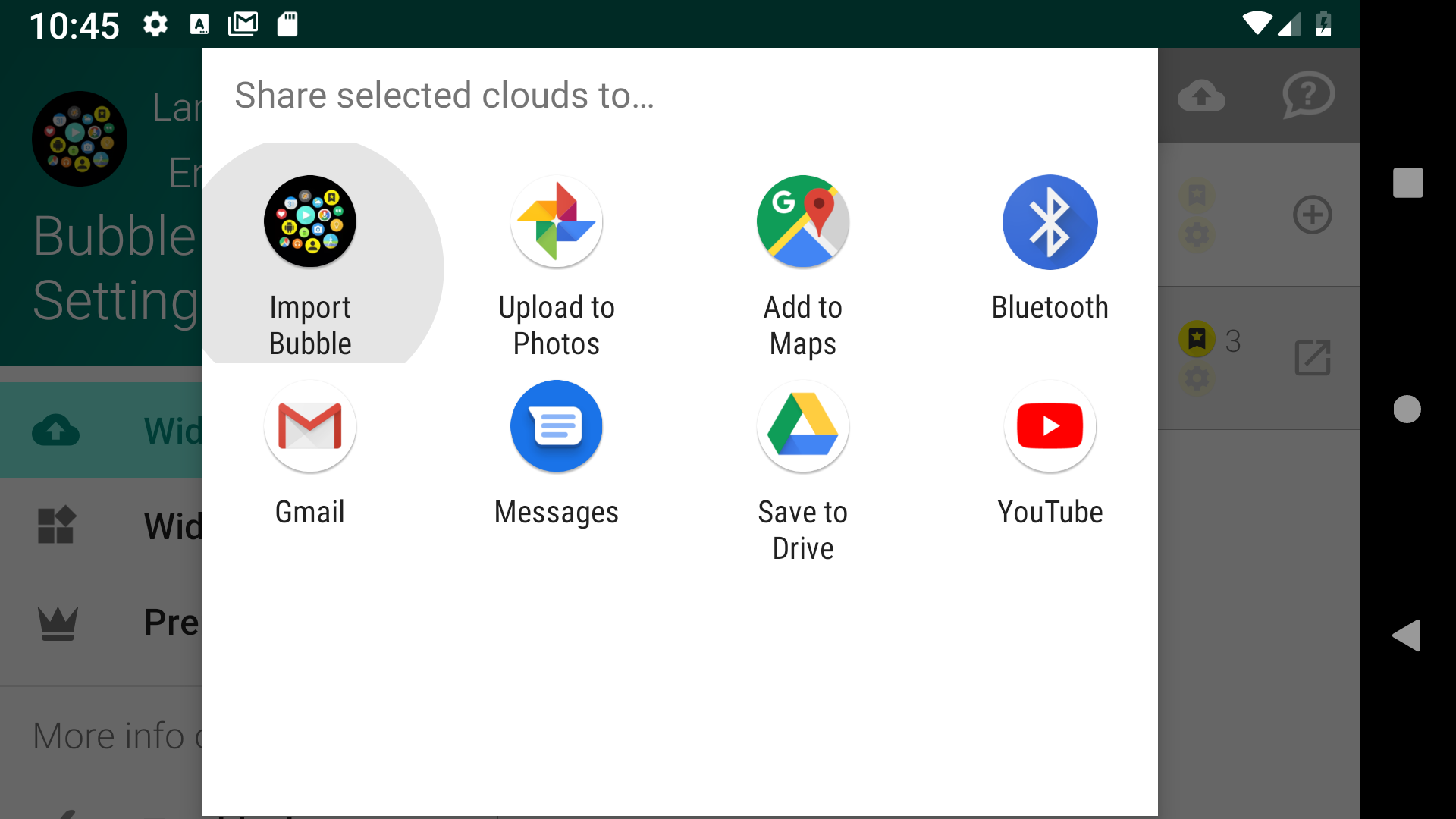The image showcases a screenshot from a mobile device, likely a tablet. The top-left corner of the screen displays the time (10:45), alongside icons for settings, mail, and SIM card status. The top-right corner shows a full Wi-Fi signal, a partial data signal, and a battery icon indicating less than half charge. 

Prominently featured in the center of the screen is a white dialog box with the header "Share selected clouds to:" followed by various sharing options. These options include:

- **Import Bubble**: Represented by a black circle with multiple icons inside.
- **Upload to Photos**: Indicated with the Google Photos icon.
- **Add to Maps**: Displayed with the Google Maps icon.
- **Bluetooth**: Marked by the Bluetooth icon.
- **Gmail**: Shown with the red and white envelope icon.
- **Messages**: Depicted with the blue speech bubble icon.
- **Save to Drive**: Illustrated with the Google Drive icon.
- **YouTube**: Identified by the red YouTube play button icon.

The screen's right-hand side contains a black vertical toolbar with buttons for "Back," "Exit," and "Shift Tabs." In the background, partially obscured by the dialog box, there is text that includes the phrase "bubble setting."